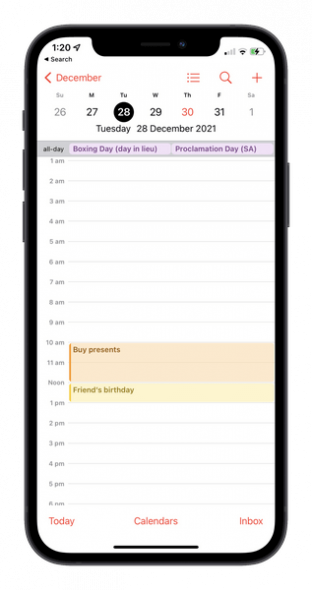This image is a detailed screenshot of a smartphone displaying the user's calendar and status information. The time is 1:20 PM, and the phone's battery is at 50%, with very weak signal reception. The date shown is Tuesday, December 28, 2021. The calendar is busy for the entire day, with specific events marked in hourly segments. The schedule starts at 1 AM and lists two major activities: from 10 AM to 12 PM, the user is set to buy presents, and from 12 PM to 1 PM, they have a friend's birthday event, possibly indicating a lunch outing. At the bottom of the screen, the calendar display options are visible, marked as 'Today,' 'Calendar,' and 'Inbox.' The phone itself is a black-colored device, making the screenshot appear as though it is directly captured from within the phone.